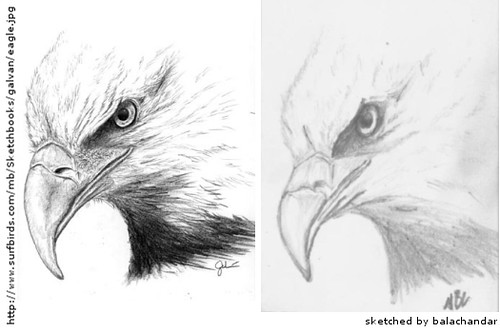The image showcases two side-by-side illustrations of American bald eagle heads, with both drawings captioned "sketched by Balachandar" at the bottom. The left eagle is meticulously detailed with well-defined shading, creating a striking and lifelike representation, while the right eagle appears less refined, akin to something drawn by a young child. The website "https://www.surfbirds.com" is displayed along the side of the picture.